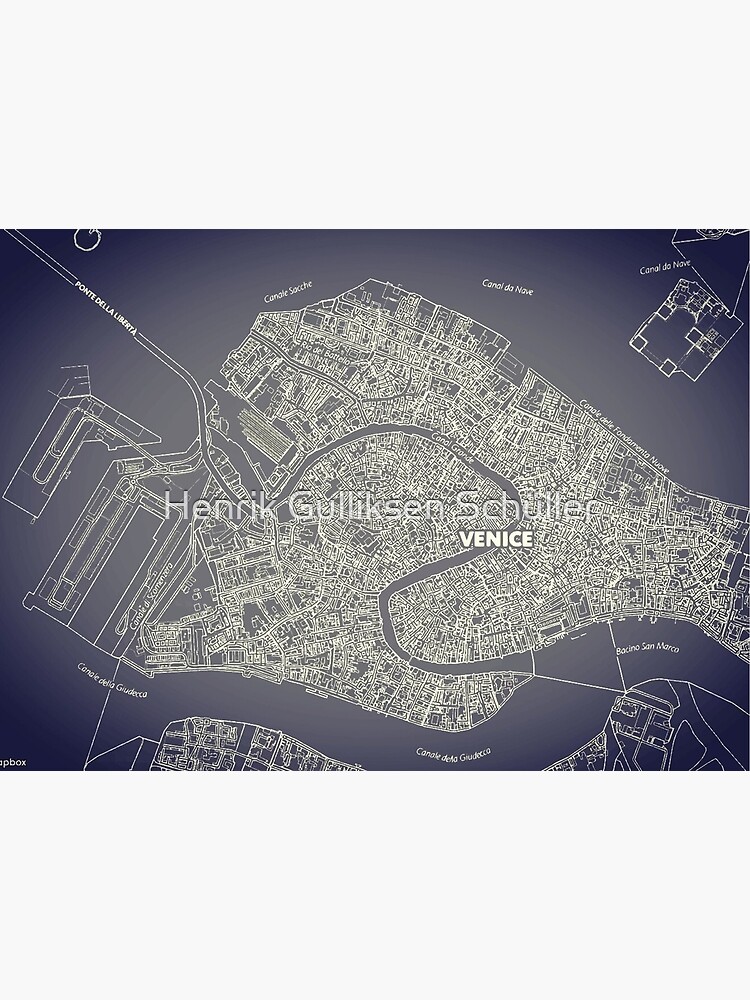This intricate and highly detailed black-and-white aerial architectural drawing depicts a map of Venice. The background of the map is rendered in dark gray, etched with delicate white lines illustrating the city's crowded and interconnected streets and canals. The canals weave through the dense urban fabric like a spider web, creating a complex but identifiable pattern. Prominent text in the center of the image reads "Henrik Gullikson Schuller," with "Venice" written below it in white bubble letters. The map includes labeled locations such as "Ponte della Libertà," "Canal Soce," "Canal da Nave," "Bassino San Marco," and "Canal della Giudecca," although the writing is small and may be challenging to read. A large river flows along the bottom of the map, connecting two land masses, and docks are visible on the left side. Despite the intricacy and minute details, the overall image is clearly illuminated, making the city's structure and waterways discernible.